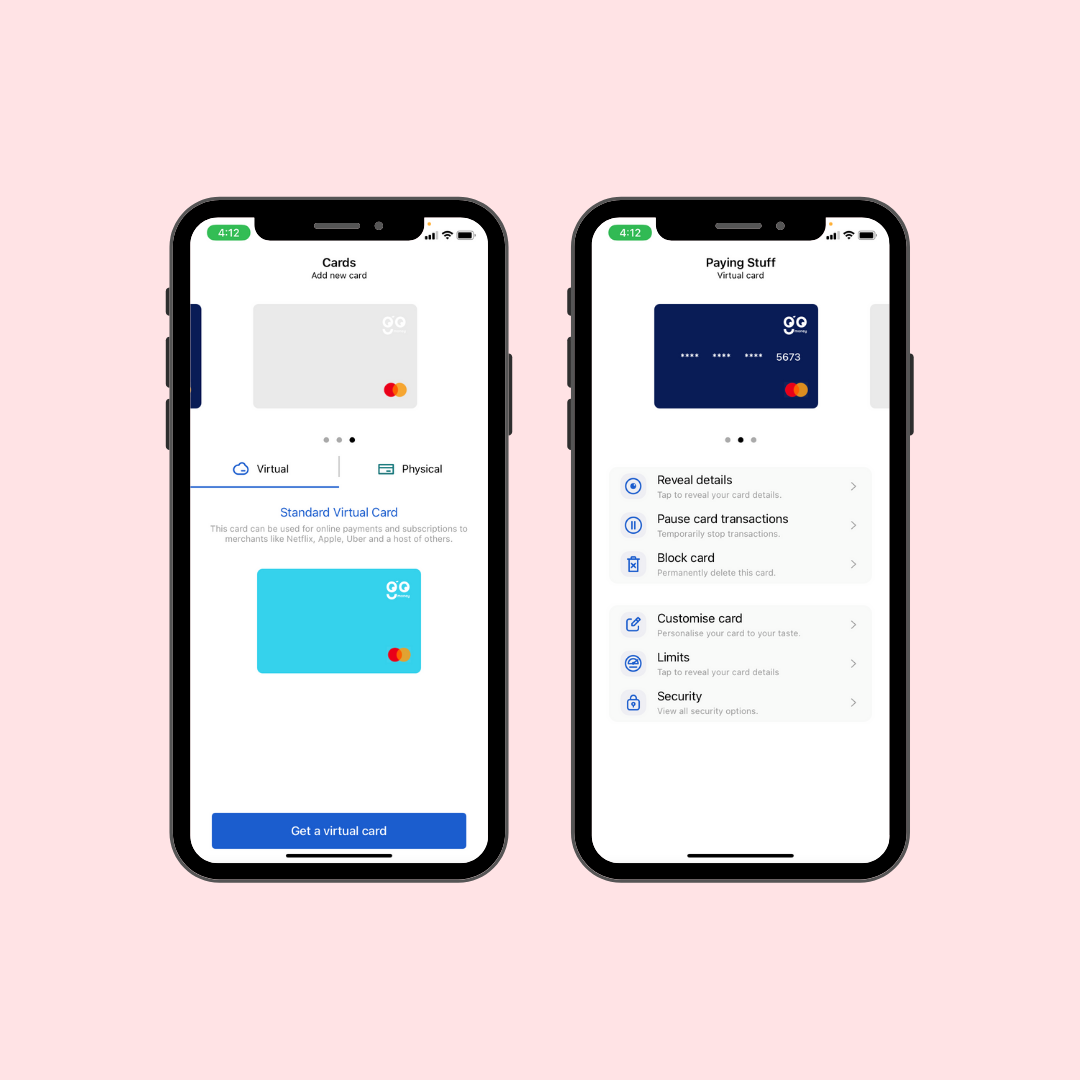The image features a pink background with two smartphones placed next to each other, both displaying similar screens from a banking app. Each screen appears to be showcasing different functionalities related to credit or banking cards.

On the left phone screen, the header section highlights a bolded "Cards" title. Immediately below this, an option labeled "Add New Card" is present, followed by a whiteish-grey rectangular placeholder symbolizing a mobile version of a credit card. This placeholder is intended for users to add another card to their account. Below the placeholder, three dots indicate the existence of multiple cards that can be swiped through. The screen differentiates between "Virtual" and "Physical" cards, with a section mentioning a "Standard Virtual Card," emphasizing its utility for online payments. Further below, there's a sequence including a light blue card and a dark blue rectangular button prompting the user to "Get the Virtual Card."

On the right phone screen, the same banking app is displayed but focuses on a different aspect of credit card management. The header reads "Paying Stuff," followed by a "Virtual Card" label beneath. This screen shows the second card in the list, represented by a filled-out dark blue credit card that reveals only the last four digits. Consistently, the three dots at the bottom of the screen suggest multiple swipable cards. The card on display comes with a set of options for the user, including revealing card details, pausing transactions, blocking the card, customizing card features, managing spending limits, and tweaking security settings.

Overall, the image presents a detailed view of a banking app’s interface specifically designed for card management, offering a range of functionalities visible on both phone screens.